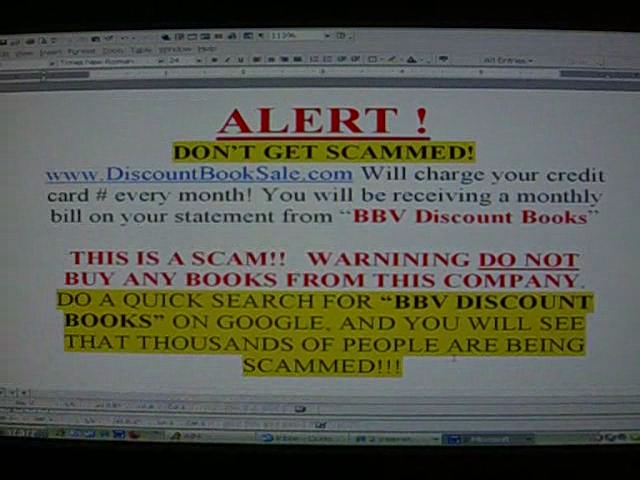The image appears to be a dim and slightly hazy screenshot of a Microsoft Word document displayed on a computer screen. The document contains several warning messages about a potential scam. At the top of the document, "ALERT!" is written in red, underlined, and prominently emphasized with an exclamation point. Below this, in black text highlighted in yellow, is the phrase "Don't get scammed." The document warns that the website "www.discountbooksale.com" will charge your credit card every month, with the statement showing charges under the name "BBV Discount Books." Following this information, in red text, it states emphatically, "THIS IS A SCAM. WARNING: DO NOT BUY ANY BOOKS FROM THIS COMPANY." Finally, in black text again, highlighted in yellow, it advises to "do a quick search for BBV Discount Books on Google and you will see that thousands of people are being scammed." This image serves as a cautionary notice to prevent others from falling victim to this fraudulent scheme.